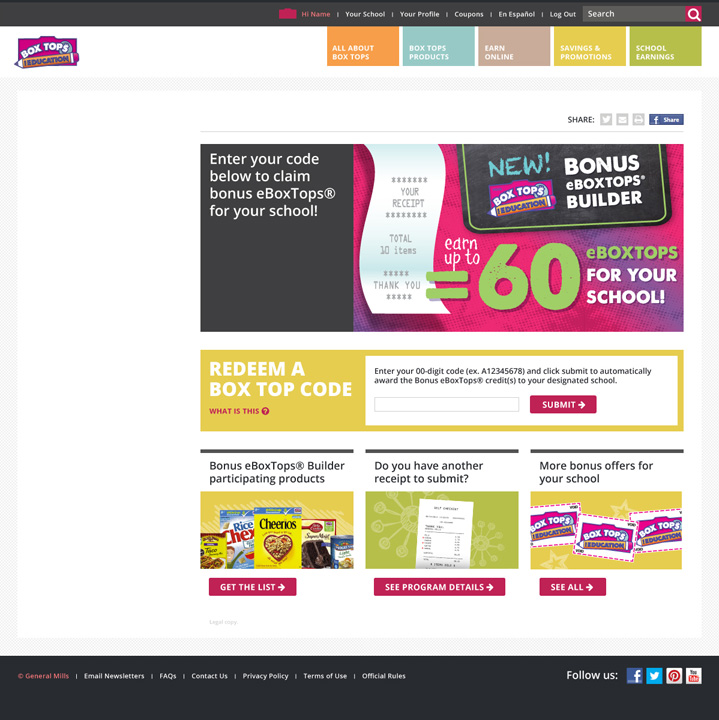The webpage features a prominent black banner at the top and bottom. The website is associated with Box Tops for Schools, recognizable by the logo displayed. This program allows users to submit box tops to earn money for their schools. 

At the top black banner, several options are available: "My Name," "Your School," "Your Profile," "Coupons," "En Español," "Log Out," and a search icon represented by a magnifying glass. Below this bar, "SHARE" is written in all caps in black print, with various sharing options including Tweet, Print, Email, and Facebook.

Further down, there's an image instructing users to "Enter your code below to claim bonus e-Box Tops for your school." Accompanying this is a small picture of a receipt and text promoting a "New Bonus e-Box Tops Builder," stating that users can earn up to 60 e-Box Tops for their school. Below this information, a yellow box prompts users with "Redeem a Box Top Code," followed by a white input field where users can type their code and click "Submit" to redeem their e-Box Tops.